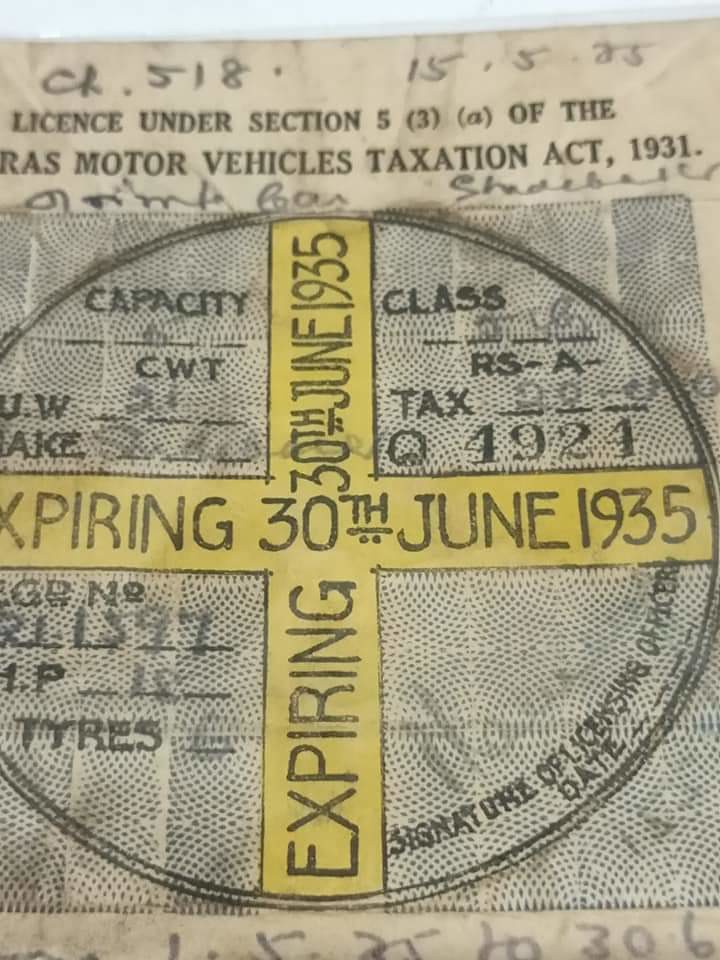This image displays an old, creased, and smudged document related to vehicle licensing. At the top, it bears the heading "License under Section 5(3)(a) of the RAS Motor Vehicles Taxation Act, 1931," flanked by handwritten notes such as "CH 518 15 575." In the center, the document features a circular emblem with a blue and grey dotted pattern. Inside this circle, there's a yellow cross, both intersecting lines of which prominently display "expiring 30th June 1935" vertically and horizontally.

Each quadrant of the circle contains specific details; the upper left mentions "capacity 15 CWT," while the upper right lists "class" and "RSA text" followed by some numbers. The bottom left corner has partially visible text including "tires," whereas the bottom right includes a footnote with the "signature of licensing officer" and "date."

Despite some cut-off sections, additional handwritten notes are visible at both the top and bottom of the document, contributing to its aged and well-used appearance.